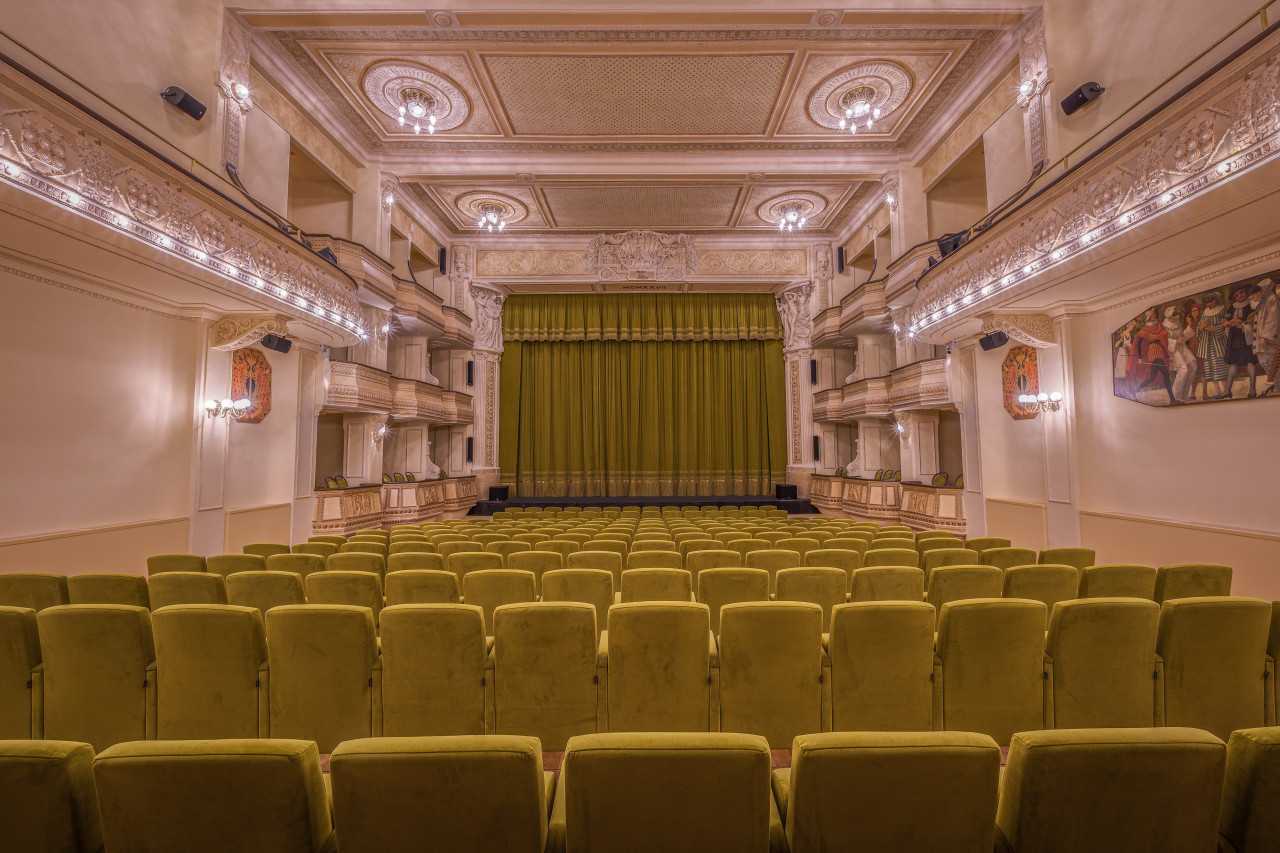This photograph captures the interior of a well-lit, empty theater viewed from the back row. The seating is arranged in multiple rows of yellowish, cushioned chairs that blend into the distance, creating an intimate yet expansive feeling. The stage, located at the front, boasts a set of closed curtains that are a harmonious mix of green-tan-yellow tones, aligned with the color of the chairs. The stage itself is a contrasting deep blue, enhancing the visual appeal.

Flanking the stage are light pink or white walls adorned with paintings and art pieces, adding an element of sophistication. The theater features tiered seating, including balconies situated on both the left and right walls, offering additional vantage points closer to the stage. Prominent on the ceiling are four grand chandelier-style lights that flood the space with illumination, along with other ceiling and wall-mounted lights enhancing the venue's brightness.

Speakers are strategically positioned around the theater, including prominent ones on the top right and left corners and more along the walls below the balconies. The overall ambiance presents a picturesque and inviting environment, ideal for enjoying a performance.